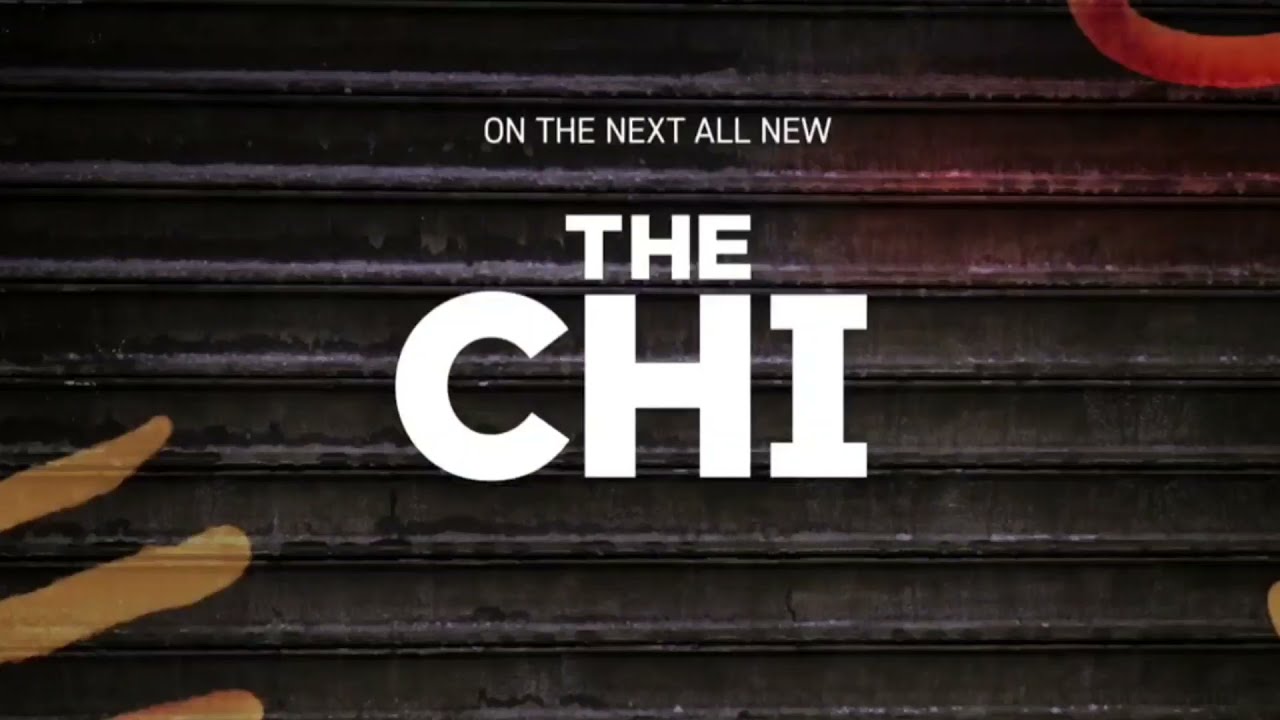The image appears to be an advertisement or a promotional still for a TV show or podcast titled "The Chai." It features a steel shutter door, akin to those used to close storefronts in urban areas, painted in a dark, gunmetal gray. The backdrop includes graffiti-like elements, with three gold streaks on the bottom left and a red half-circle on the upper right, partially reflected onto the shutter. The primary focus is the text: "On the next all-new" in smaller writing, with "The Chai" prominently superimposed in large white font at the center. The overall scene sets a gritty, urban tone, likely hinting at the show's thematic connection to Chicago.